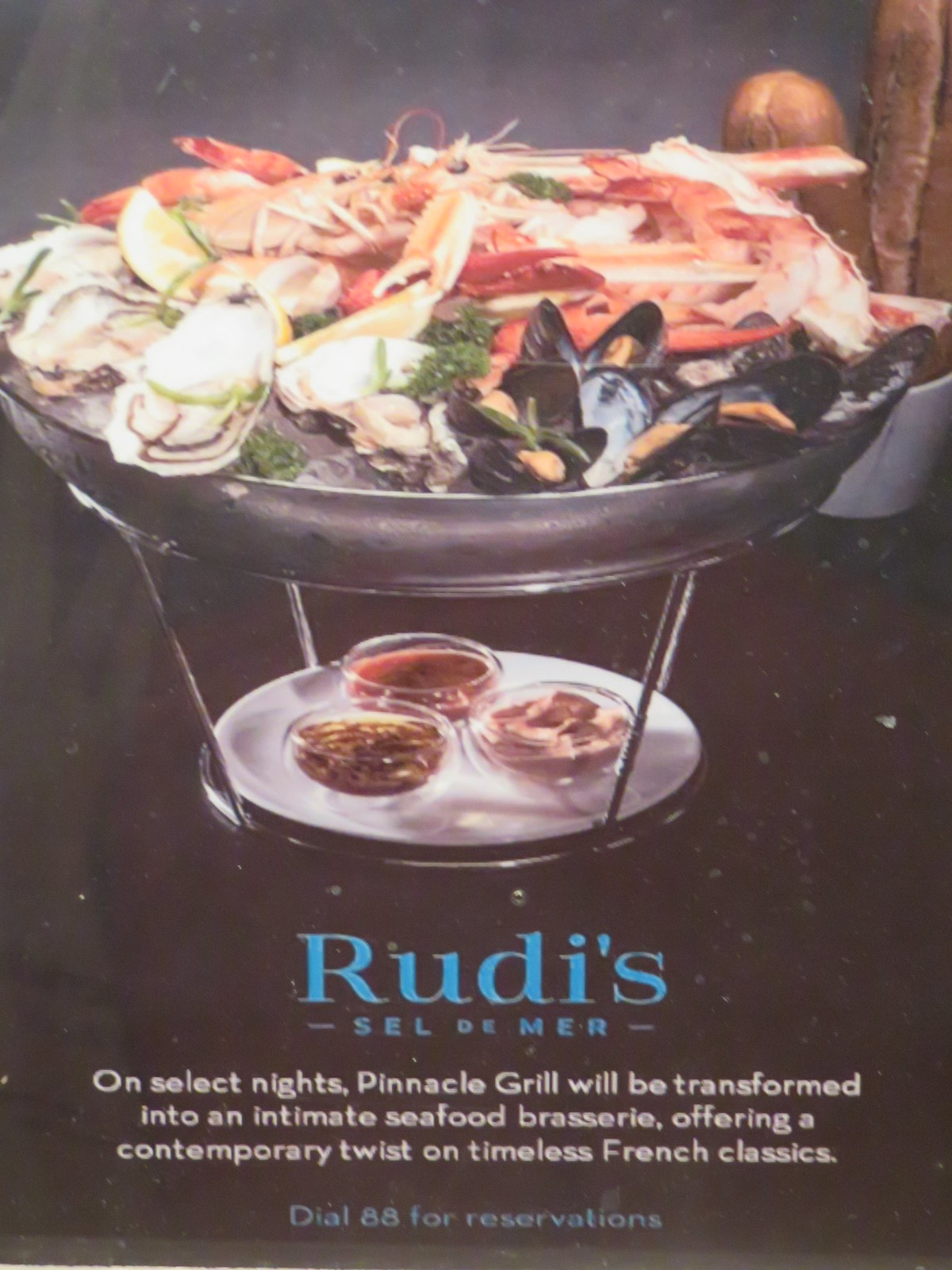This is a tall rectangular image featuring an advertisement for a restaurant, possibly located in a hotel lobby. At the top of the image, set against a dark surface with a gray background, there is a silver bowl on a silver stand, with a white saucer below that holds three clear ramekins of various sauces: one reddish, one brownish-yellow, and one pinkish-white. The silver bowl brims with an assortment of seafood, including shelled items, shrimp, mussels, crab legs, lobster tails, oysters, clams, lemons, and green garnishes drizzled with sauces. In the top right corner, nearly out of view, there is a bowl of bread. At the bottom of the image, in bright blue text, it reads "Rudy's Sel de Mer." Beneath that, in white text, it states, "On select nights, Pinnacle Grill will be transformed into an intimate seafood brasserie, offering a contemporary twist on timeless French classics." Finally, in blue text, it adds, "Dial 88 for reservations."